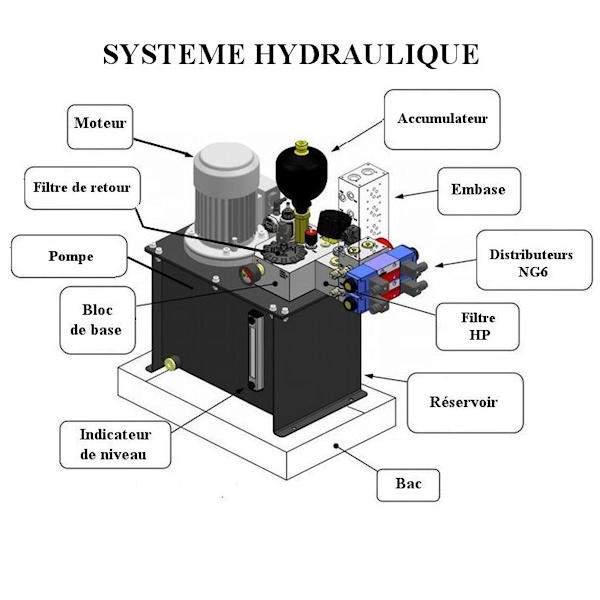The image is a detailed diagram of a hydraulic system, labeled in French, with the title "SYSTEME HYDRAULIQUE" at the top in bold, black, all-caps letters against a white background. The central machine consists of a dark gray rectangular body with a cylindrical shape on top. Key components are identified with white, black-bordered text boxes and arrows. The labeled parts include:

1. **MOTEUR**: The motor, with a black arrow pointing to the cylindrical shape on top of the rectangular body.
2. **ACCUMULATEUR**: Shaded in black, located to the right of the cylindrical motor.
3. **EMBASE**: A cubical shape below the Accumulateur.
4. **DISTRIBUTEUR NG6**: A blue, red, and gray piece on the far right.
5. **FILTRE HP**: A gray square piece next to the Distributeur NG6.
6. **RÉSERVOIR**: Pointing to the large dark gray base of the machine.
7. **BAC**: A white base beneath the large gray base, likely the drain plug.
8. **INDICATEUR DE NIVEAU**: Located on the left side, pointing to smaller parts.
9. **BLOC DE BASE**: Another component on the left side.
10. **POMPE**: Indicating the pump.
11. **FILTRE DE RETOUR**: Labeling the return filter.

This comprehensive labeling guides the viewer through the various vital components of the hydraulic system.